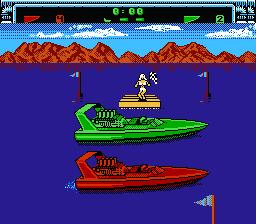In this image from a video game, we see a vibrant scene set amidst vast expanses of water. Two speedboats, one red and one green, are side-by-side, poised at the starting line for an upcoming race. A woman stands on a small floating dock in the middle of the ocean, holding a checkered black-and-white flag high, ready to signal the beginning of the race. Surrounding her are two anchors and marker buoys that define the race course. In the backdrop, majestic reddish mountains rise against the horizon, under a brilliant turquoise sky dotted with clouds. A time strip, rendered in neon green, stretches across the top of the image, flanked by red icons on the left and green icons on the right, adding to the dynamic visual elements that set the stage for the thrilling aquatic race.